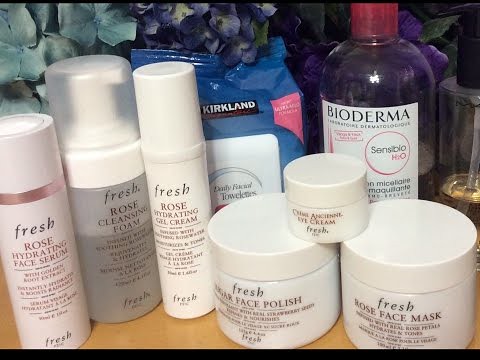A curated collection of personal care products is meticulously arranged on a light, natural wooden surface. Framed by a subtle black border at the bottom, the scene is accented with delicate blue and purple hydrangea blooms, mainly clustered in the upper left and center, with a singular flower visible on the right. Dominating the ensemble are several cylindrical bottles from the Fresh brand, distinguished by their white tops. In the background, a package of Kirkland brand daily facial towelettes, encased in a blue plastic bag, subtly peeks out. To the right, a clear plastic bottle of Bioderma micellar water, capped with a vibrant pink top, adds a splash of color. The products prominently displayed in the foreground encompass Fresh Rose Hydrating Face Serum, Fresh Rose Cleansing Foam, Fresh Rose Hydrating Gel Cream, Fresh Sugar Face Polish, an unidentified eye cream by Fresh, and Fresh Rose Face Mask.